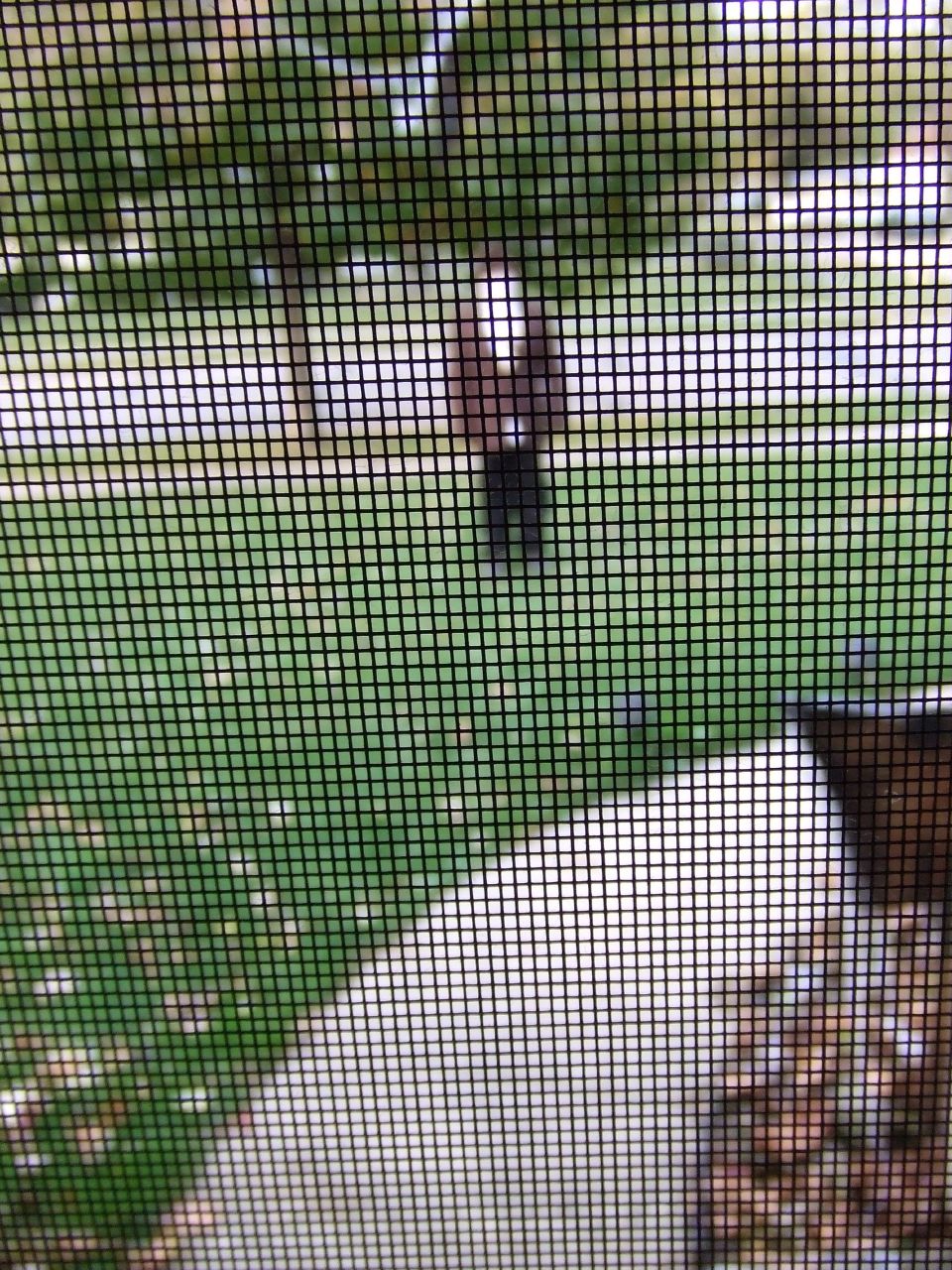In this color vertical photograph, taken through a black screen door or window, the dominant feature is the screen itself, covering the entire image with a grid of little black squares. Beyond the screen, the scene depicts a front yard bathed in daylight. A gray sidewalk curves to the right from the bottom of the image, bordered by green grass on the left and a garden bed of rocks and pebbles in various shades of black, gray, white, and tan on the right. Two black solar lights line the top of the walkway as it prepares to turn.

Standing in the grass, facing toward the screen, is a person with brown hair (or possibly a brown hat), dressed in a white shirt layered with a long-sleeved brown shirt or jacket and black pants. Behind this figure lies another straight sidewalk, more grass, a large tree, a street, and finally another grassy area behind the road. Sparse flowers dot the lower left lawn, suggesting it might be fall. The overall scene is brightly lit, indicating it is daytime.